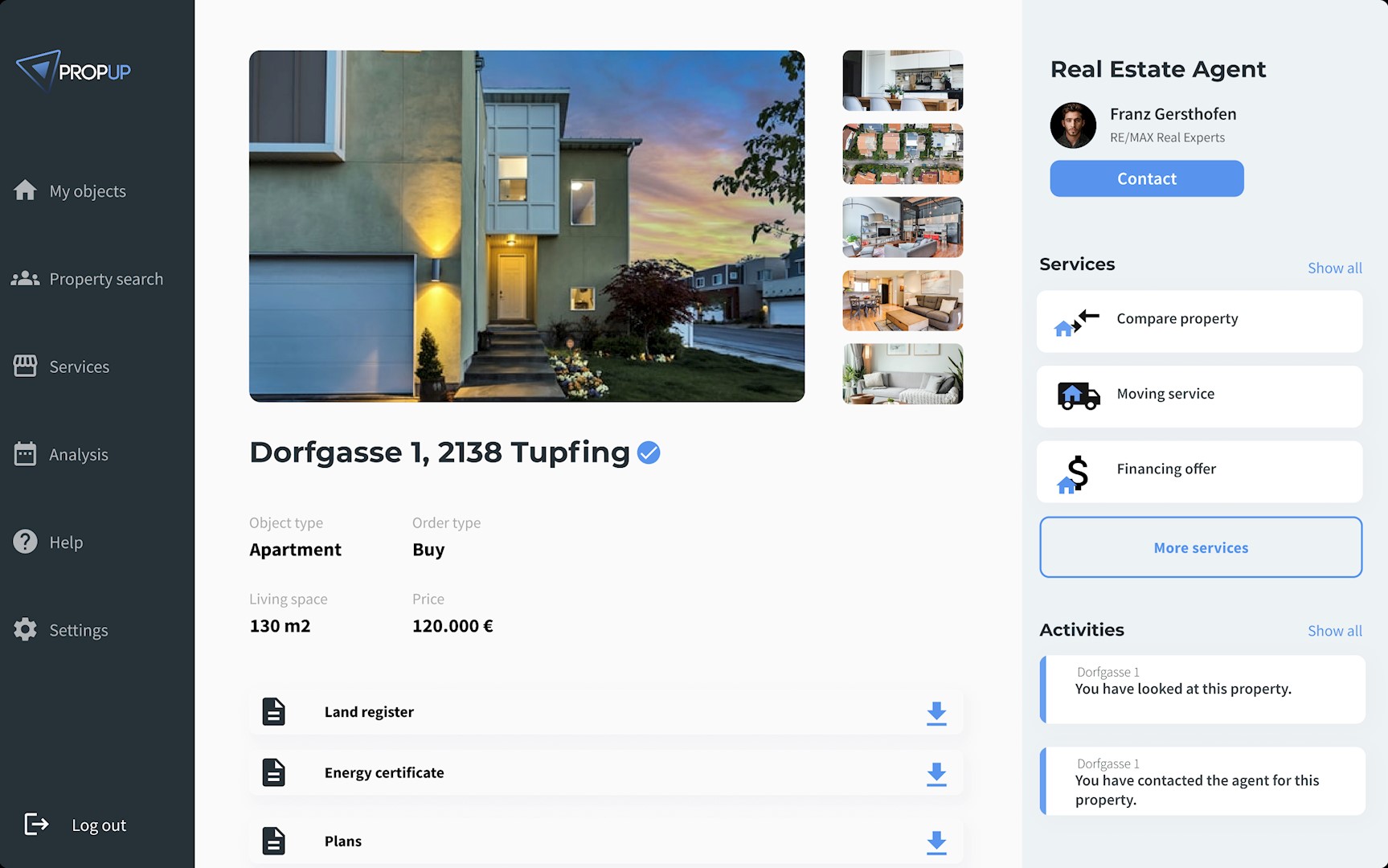**Caption:**

The interface displays a vertical column on the left with tabs labeled: "Prop Up," "My Objects," "Properties," "Services," "Analysis," "Help," "Settings," and "Logout." The main image showcases a stone building with a prominent garage door at the front. Above the garage door, there's an exterior light fixture. The building also features a set of steps leading up to the main entrance door. Surrounding the property, there's a well-manicured grass lawn and a large tree. The scene extends to show a road in the foreground. In the backdrop, clouds are visible in various shades of blue, yellow, and red.

On the right side of the image, there is a list containing numbers and descriptions: "1, 2, 3, 4, 5," "pictures," "door," "gas," "1, 2, 1, 3," and "tough machine." Furthermore, the information specifies "Hydrotech Apartment, Order Type 5," which signifies it's a living space with the listed features. The property is priced at $120,000. Additional details such as "language," "short energy," and "2k plants" are also mentioned.

Devices are tagged with "real estate agent," "friends," "guests," "often," and "aria/max," indicating possible communication methods or statuses. Under "real experts," options like "services," "compare property," "movement service," and "financing offer" are listed. A highlighted rectangle labeled "more services" appears with further specifics noted below, such as "activity" and references to interactions like, "each wall," "door for gas," and "you have looked at this property." The system also records that "you have contacted the agent for this property." The overall background features are stated as "grey" and "white."